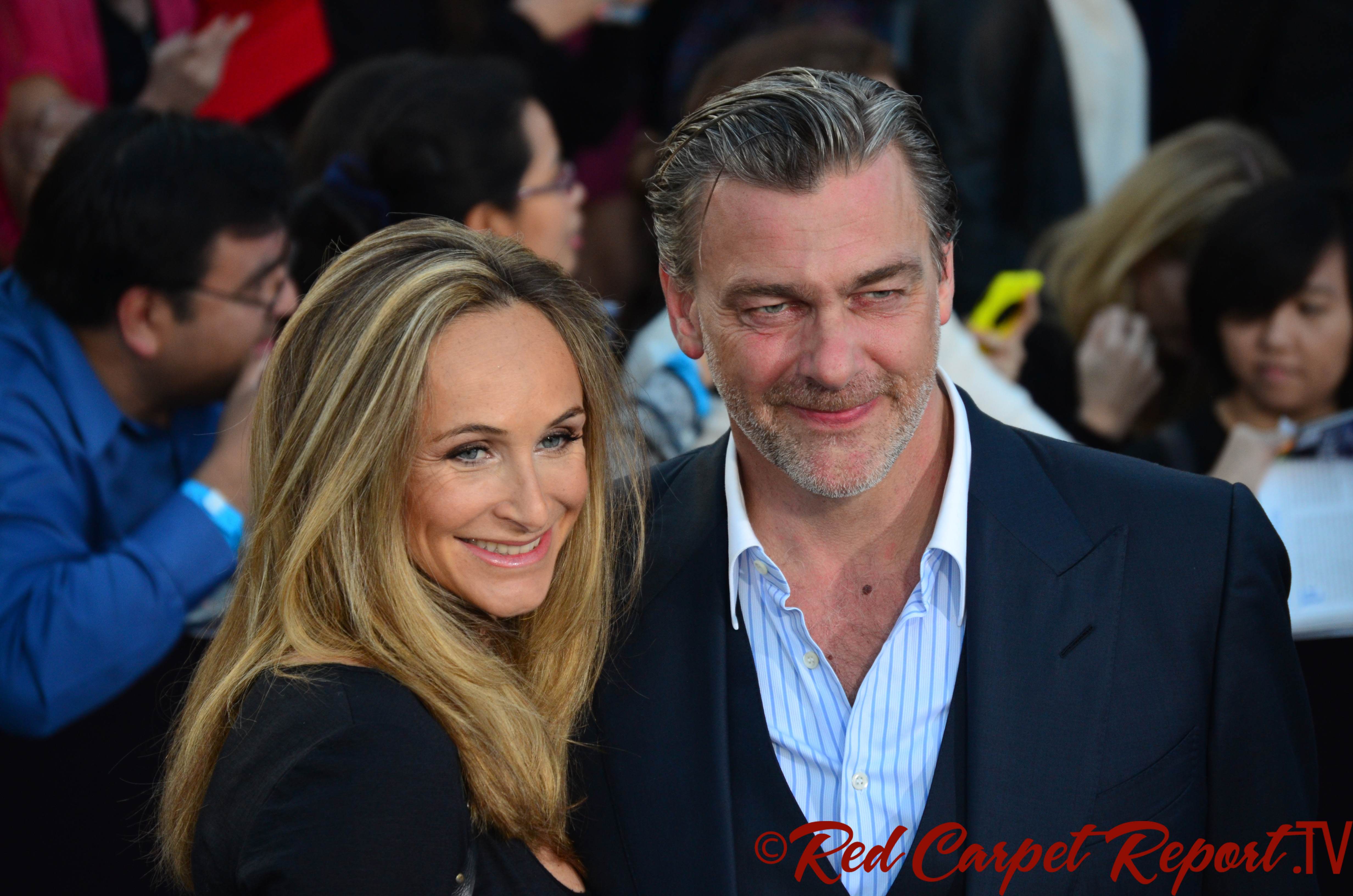In this detailed image, the lower right-hand corner features the cursive, red text "copyright red carpet report dot TV" with the letters "TV" unitalicized. The focal point of the image showcases two people, a man, and a woman, both smiling and appearing to enjoy the moment on what is presumably a red carpet, as indicated by the text.

The woman stands to the left, sporting long blonde hair that falls to her shoulder blade level. She is dressed in a black suit or dark blouse, visible from just above her head to slightly below the chest. Facing the man with her body, her face is turned forward, radiating a cheerful smile and showing off her blue eyes.

Next to her, the man, who is also smiling, faces directly forward. He is dressed in a dark blue suit with a white and blue pinstripe shirt, part of which reveals a bit of chest hair. His graying beard complements his slicked-back, short gray hair. The interactions suggest he might be holding the woman gently.

In the background, there is a crowd of fans and photographers, indicating the ambiance of a red carpet event. A woman on the right side of the frame is seen whispering to another person, while another man in a dark blue shirt gazes off to the right, seemingly interested in something outside the main subjects of the photograph.